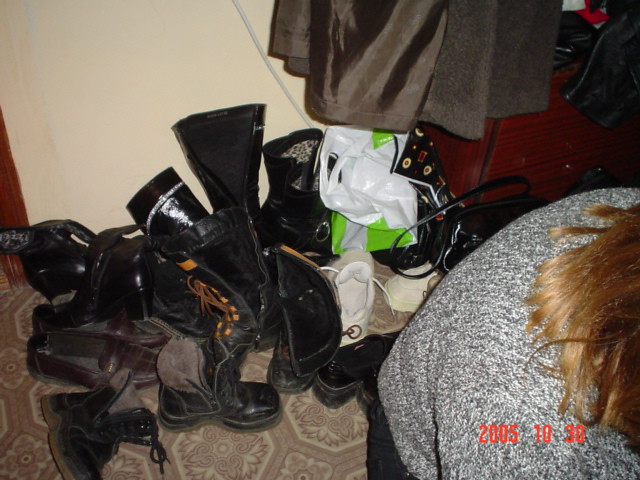The image is an indoor snapshot taken on October 30, 2005, as indicated by the date "2005-10-30" written in orange text in the lower right-hand corner. In the foreground, a person with short, dirty blonde hair, which reaches their shoulders, is visible. They are wearing a variegated gray and cream sweater along with dark pants. The individual appears to be bent over or squatting, partially covering the area rug behind them. The rug features a beige and cream design with hexagons and squares containing floral prints.

Scattered on top of this rug is a jumble of mostly black shoes, predominantly boots of various lengths, with some high heels and possibly a white sneaker. A plastic shopping bag sits amidst the shoes, and the bottom hem of a coat is visible hanging at the top of the image. A red-brown wooden chest of drawers is also present in the background. The overall scene suggests a casual moment inside a home, capturing the clutter of shoes against the backdrop of a intricately designed rug and household furnishings.